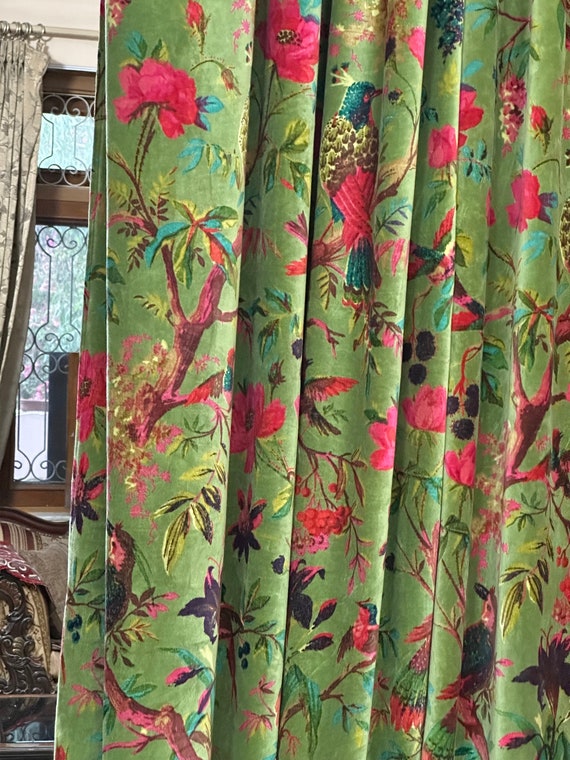The image depicts a vibrant, tropical-themed curtain made from a green, creased fabric that dominates the frame from top to bottom. The curtain is adorned with an intricate pattern featuring red vines, green and red foliage, and red flowers with yellow and black-dotted bulbs. Birds of various colorful plumages populate the scene, including birds with dark red and pink feathers, lighter red and brown hues, and one bird prominently featuring a blue head with tufted feathers, yellow, pink, and blue plumage on its back. The motif includes tree limbs and branches in shades of brown. Behind the curtain, a window with decorative ironwork sporting bone-like formations provides a glimpse into the adjacent room. The window's metal gates are curved at both the top and bottom, and beyond it, elements of the room, such as a chair and possibly a sofa and coffee table, are partially visible.